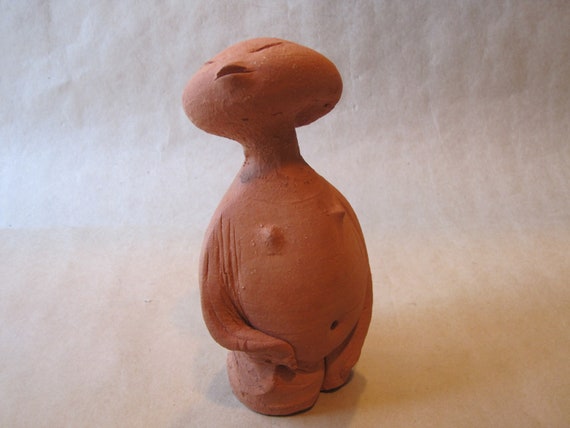The image captures an intricately detailed, almost human-like statue made of red clay with an orange hue. This stylized sculpture stands upright on an off-white, almost beige, sheet of paper, which serves to neutralize the background. The statue has an oblong, vertically positioned head with a small, slightly beak-like open mouth and two lines representing closed or squinted eyes, conveying a sense of contemplation. The neck is slender, and the torso features a round belly with a visible navel and two prominent nipples. The statue's slim arms lack detailed hands but one arm appears to rest on its hip while the other is not visible. The figure casts a slight shadow to the right, creating depth, and seems to be gazing towards the upper left corner, adding a mystical, otherworldly aura to the piece.